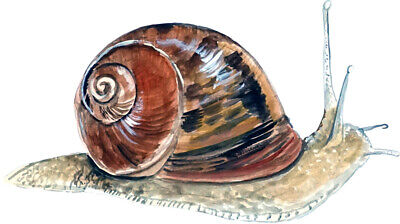This painting depicts a snail against a stark white background, with the snail occupying most of the frame. The snail is heading towards the right, featuring two distinct antennae standing upright and two smaller feelers extending horizontally in front of its head. The snail's body exhibits a mottled gray-and-tan coloration, with a more pronounced tan near the head and a grayer hue towards the tail, possibly delineated with pencil marks and enhanced by small vertical hatch marks on its lighter underbelly. Its large, spiraled shell, characterized by its shiny surface, swirls prominently, showcasing rich brown tones intermixed with medium brown areas and dark black spots. The center of the spiral is positioned near the rear of the snail, and the overall shell structure appears to be highly detailed and meticulously painted, creating a contrasting effect with the more dull and smudged appearance of the snail's body.